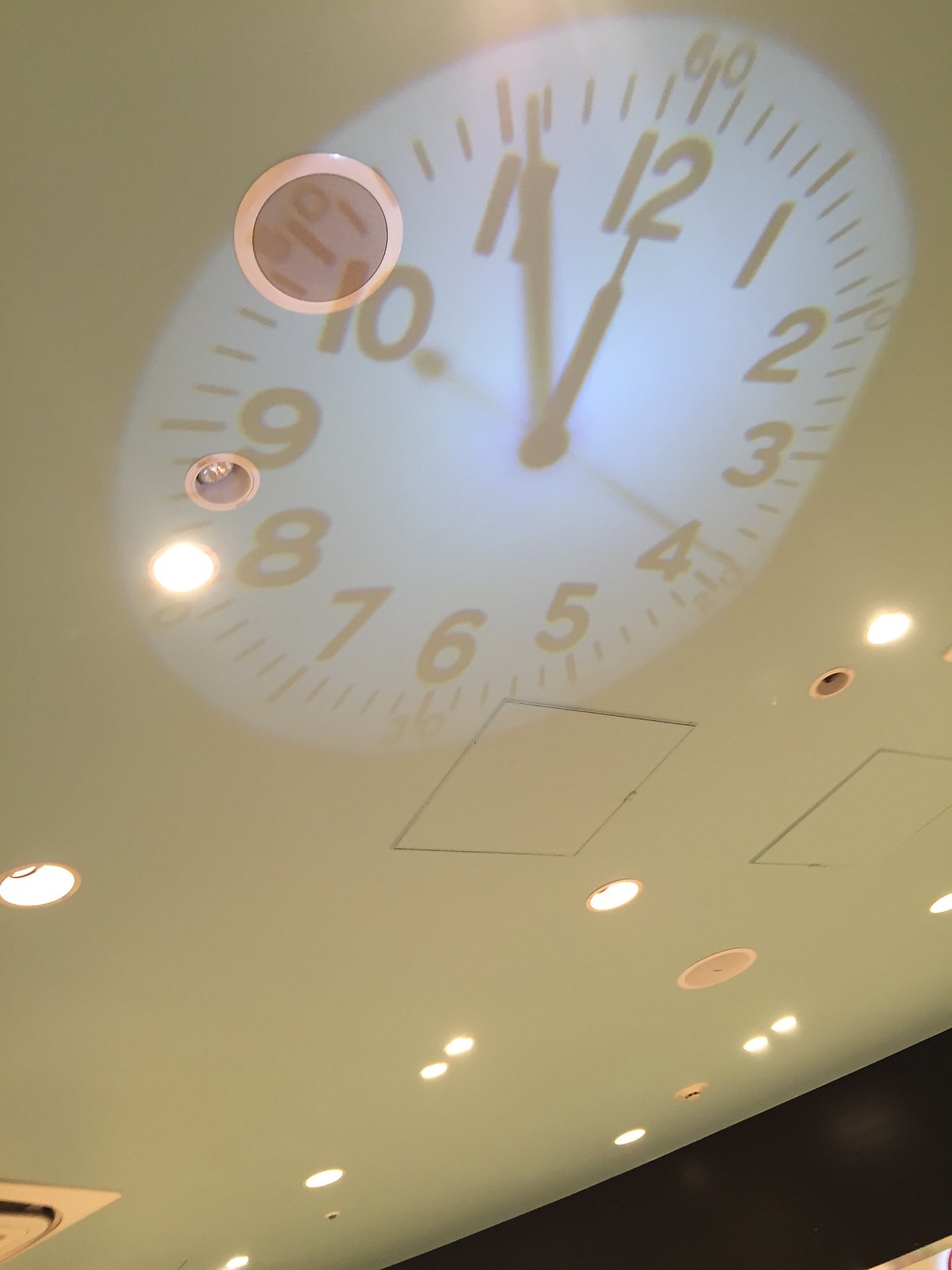The image shows a close-up view of a light-colored, likely white, ceiling of a room with several circular light bulbs recessed into it, some of which are illuminated. Projected onto the ceiling is the image of a clock, originating from a digital projector positioned below. The clock features a round white face with black numbers from 1 to 12, and three black hands indicating the time as 4 minutes to 12. In addition to the clock, the ceiling has cut-out squares that appear to be vents or possibly for other installations, and a visible speaker, suggesting an environment such as a classroom. The lower right corner of the image reveals the edge where the ceiling meets the black-painted top of the wall. The setting seems to be indoors with artificial lighting, as it appears to be dark outside.